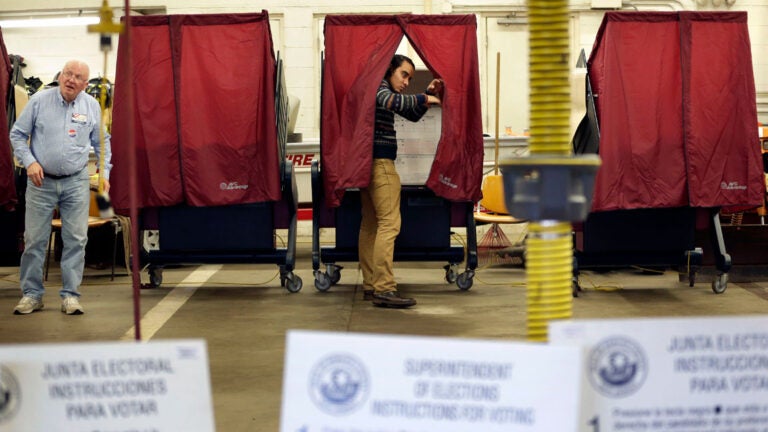The image captures the interior of a temporary voting setup within a building. Three red-curtained voting booths, each housing a machine on wheels, dominate the scene. An older man stands to the left, clad in blue jeans, a light blue button-down shirt adorned with a few stickers, and glasses. He appears to be observing something or someone outside the frame. In the middle booth, a younger man with dark hair is either entering or exiting, wearing a sweatshirt, cargo pants, and brown shoes. The other two booths are empty. The foreground features various official notices and voting papers with names on them, while a rake and some other miscellaneous items are visible in the background, hinting at the improvised nature of the space. The setup ensures privacy for voters, allowing them to cast their votes without being seen.